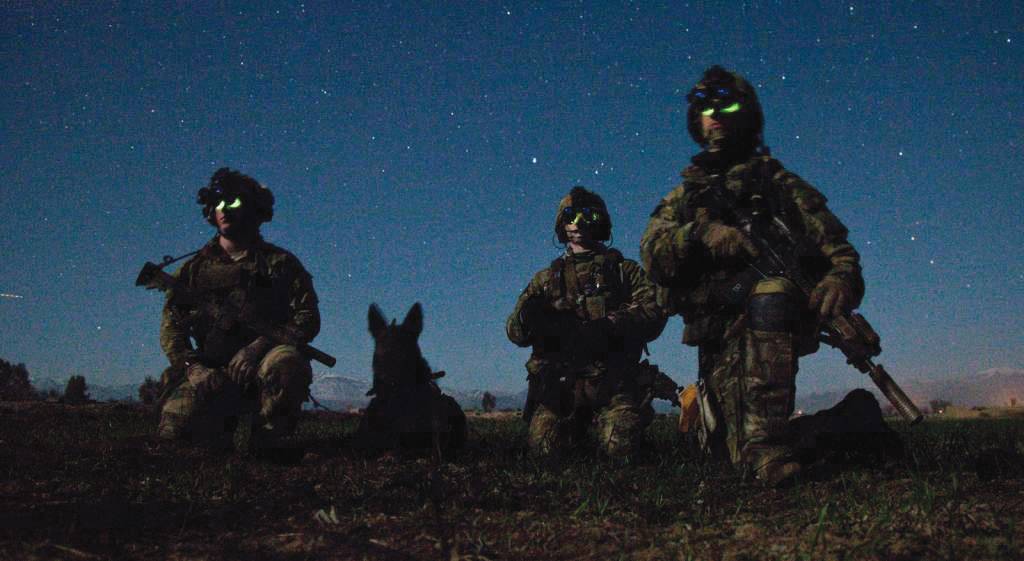In this atmospheric nighttime scene, three soldiers in tactical gear are positioned on the ground with a German Shepherd between them. The soldier on the left is crouched down with one knee up, gripping his rifle firmly in front of him, and equipped with night vision goggles and a helmet. Next to him, the German Shepherd with characteristic pointy ears rests attentively on the ground. The central soldier is kneeling with both knees on the ground, possibly holding binoculars, and is similarly dressed in military fatigues with a helmet and goggles. The soldier on the right is partially kneeling with one knee on the ground and the other foot planted, appearing slightly closer and larger in the frame. He holds his rifle at his side and also sports night vision goggles. The scene is bathed in a dark, bluish hue indicative of nighttime, with the ground appearing as a blend of dirt and grass. The backdrop features a night sky filled with dots of starlight, adding to the overall somber and vigilant mood of the image.